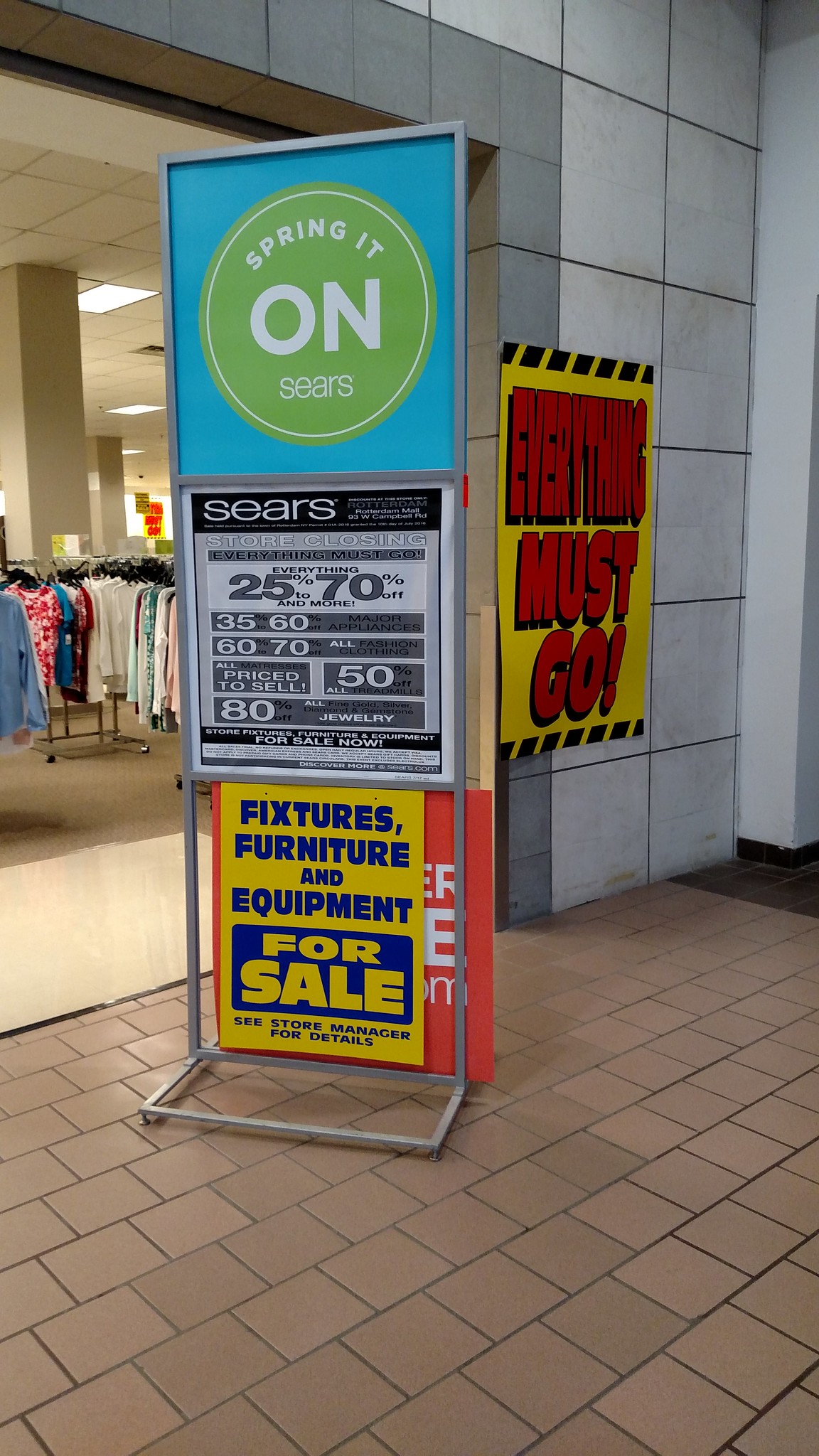The image captures a scene from a mall featuring a series of promotional signs for a Sears store. At the top is a prominent blue sign that reads "Spring it on" with the Sears logo. Below it, a green circular sign announces significant discounts, displaying "25-70% off" on various items. More specified discounts are listed as follows: "35%, 60%, 70% all reduced price to sell," and "50% off all 80% on jewelry," all in black and white text.

The bottom sign highlights that "fixtures, furniture, and equipment" are for sale and prompts interested buyers to see the store manager for more details. To the right, a bright yellow sign with bold red letters declares "Everything Must Go."

The store’s floor transitions from brown tile on the right to white tile on the left. Visible in the background are racks of women's clothing. The walls are covered in light gray tiles, adorned with smaller dark gray tiles around the archway leading to an adjacent store, which is supported by pillars.